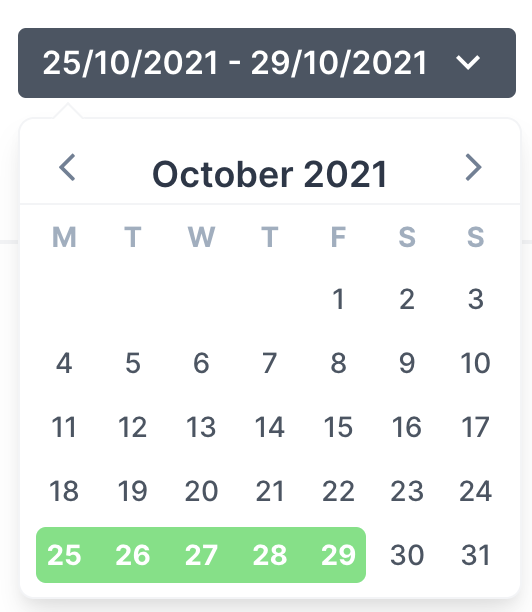A digital calendar for October 2021 is displayed, featuring a dark grey background at the top. This section prominently shows the date range "2025-10-2021 to 29-10-2021" in white text. Below, the current calendar month, October 2021, is shown with navigation buttons on either side to move to the previous or next month. The days of the week are arranged from Monday on the left to Sunday on the right. Highlighted in green are the dates from Monday, 25th to Friday, 29th, with the numbers written in white. Other dates remain unhighlighted and appear in black. The highlighted dates at the bottom match the date range displayed at the top.